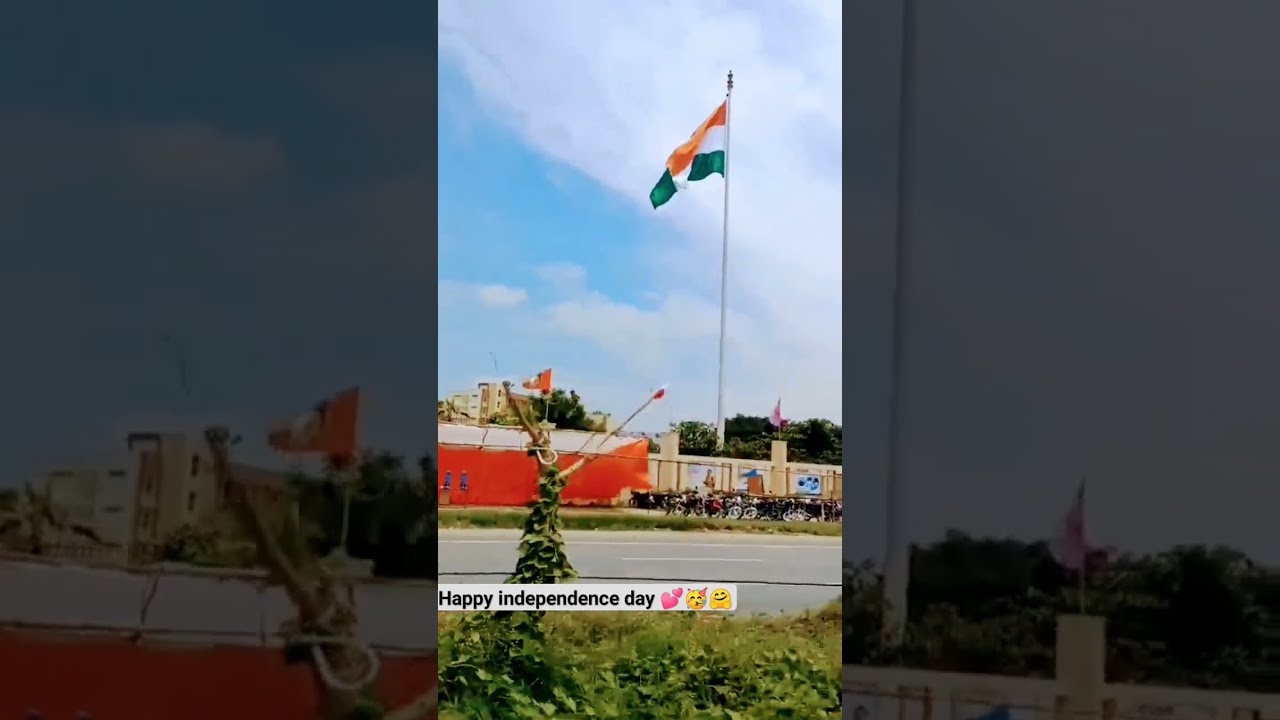The image presents a dark, underexposed photo of an outdoor scene during the day, making it challenging to discern details. At the center of this backdrop is a smaller, well-lit vertical rectangle showing a red, one-story factory-like building across the street. The sky in this inset photo is blue with wispy clouds, and the lighting is correct. 

This building features tan sections with small towers, one of which has a flagpole that prominently displays an Indian flag with horizontal stripes of orange at the top, white in the middle, and green at the bottom. In front of this building, there's a parking lot filled with lines of bicycles or motorcycles. Vegetation, such as green grass and kudzu vines, is visible in the foreground.

In the smaller, well-lit rectangle, a large flag on the right side of the image waves above the building, and there are thin clouds dispersed in the sky. This inset photo includes text stating "Happy Independence Day" followed by heart, celebration, and smile emojis, with three additional emojis near the bottom. Contrasting the dark backdrop, this central rectangle highlights a celebration theme with clear visibility of the surroundings and elements.